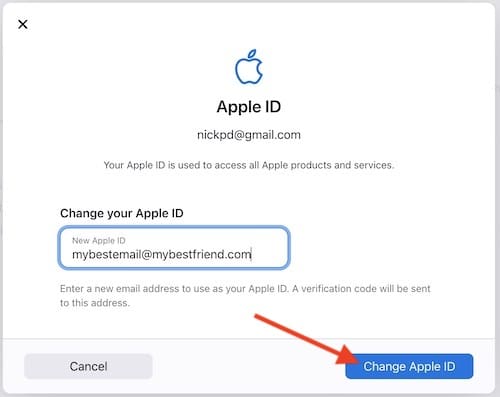**Caption:**

The image is a screenshot of an Apple ID screen, presented against a white background with a light gray border. It appears almost square in shape. Centered just below the top, the iconic Apple logo is prominently displayed. Below the logo, the text "Apple ID" is written in black font, followed by the email address "NickPD@gmail.com". Additionally, a note beneath this explains, "Your Apple ID is used to access all Apple products and services."

A section labeled "Change your Apple ID" is prominently displayed further down. Below this, there is a blue-outlined text box with the placeholder text, "New Apple ID," in small gray type. The user has entered "mybestemail@mybestfriend.com" in the text box. Underneath the input field is a brief instruction in small gray text: "Enter a new email address to use as your Apple ID. A verification code will be sent to this address."

At the upper left-hand corner, an "X" icon is available to close the window. At the bottom left part of the screen, there is a gray "Cancel" button, while a blue "Change Apple ID" button is positioned at the bottom right. A downward diagonal red arrow points from the text box where the new email is entered to the "Change Apple ID" button, emphasizing the call-to-action.

This detailed and informative layout serves to guide users through the process of updating their Apple ID on their devices.